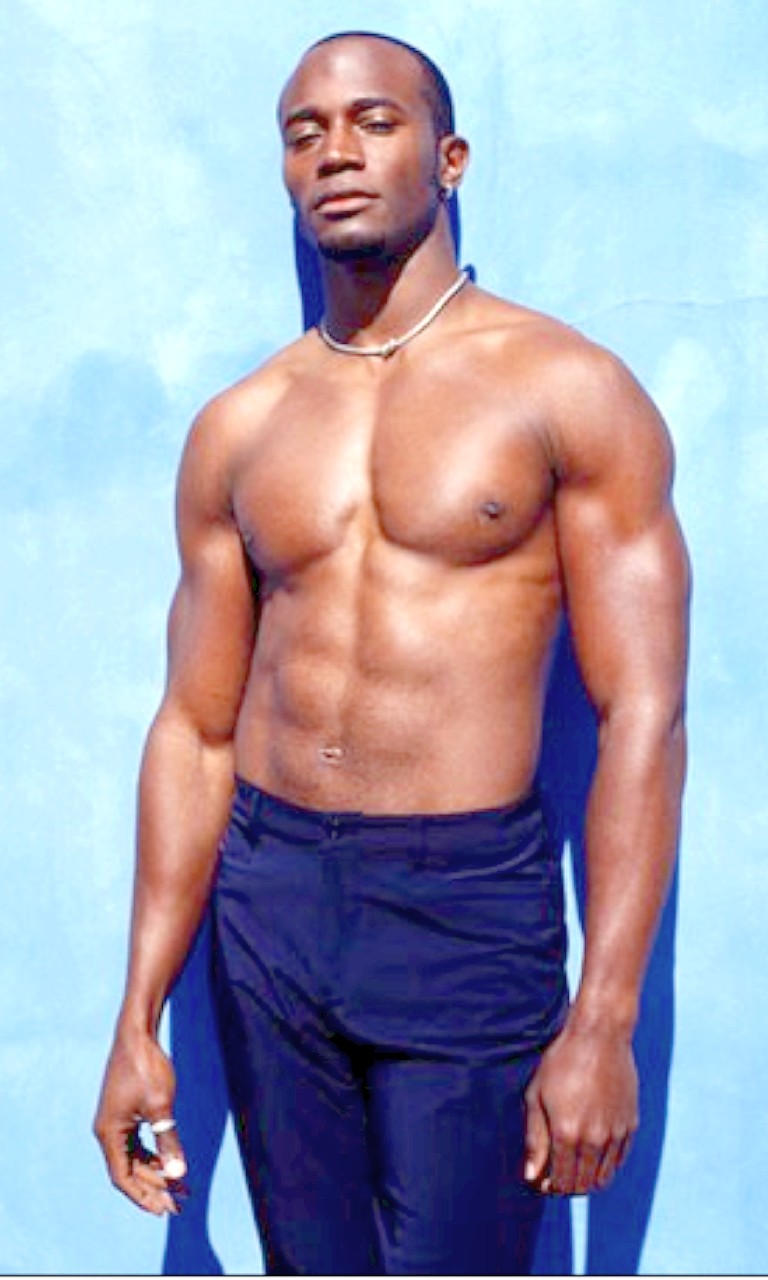This is a highly detailed photograph of an African-American man, possibly around 25 years old, standing and facing the camera. He exudes a muscular physique with defined six-pack abs and is shirtless, showcasing his well-toned upper body. His skin is dark, and he has a slight goatee under his chin while maintaining a mostly clean-shaven appearance. His hair is very short.

He is adorned with a thick silver chain featuring a knot around his neck that sits snugly, not extending far beyond his collar bones. Additionally, he wears a ring on his left thumb and an earring in his left ear. 

The man is clad in dark blue, almost navy satin-like trousers that reflect the light subtly, enhancing the overall image's aura. He stands against a light blue backdrop that resembles a cloudy sky or a watercolor painting. This artistic background amplifies the visual appeal of the photograph, with a dark blue shadow of his silhouette cast prominently behind him. The image captures not only his physical presence but also conveys a model-like poise and elegance.